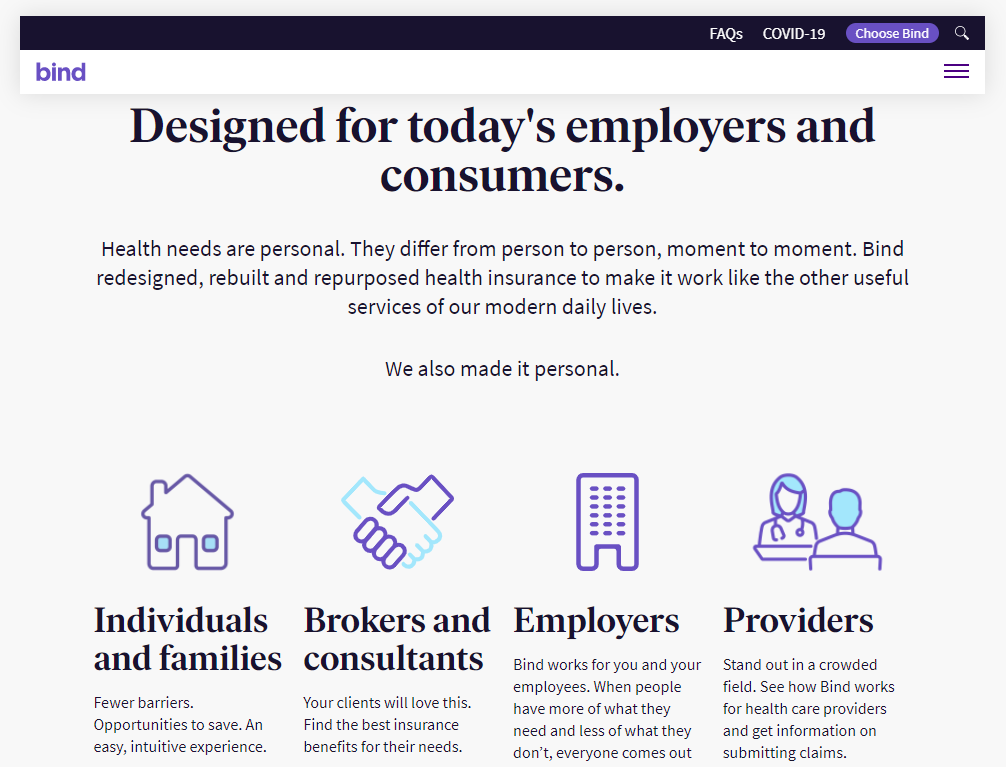The image features a detailed layout with various sections and text elements designed to provide information about Bind's health insurance services. 

At the top, the background is a deep navy blue. On the right-hand side, "FAQS" (Frequently Asked Questions) is written in white. Underneath, "COVID-19" is also displayed in white text. Below this, there is a purple oval with the phrase "Choose Bind" in white inside it, accompanied by a white search bar adjacent to it.

Next, the background transitions to white. On the left-hand side, the text "Binds MSP" is written in purple, indicating the website. Below this section, there is another area with a very light gray background. The heading within this section reads "Design for Today's Employees and Consumers" in black text. Further down, it explains, "Health Needs are Personal. They differ from person to person, moment to moment. Buy, redesign, rebuild, repurpose health insurance to make it work like the other useful services of our modern-day lives. We also made it personal."

The next part of the image features four columns, each with its own set of information:

1. **Individuals and Families**:
    - This section has an icon of a purple house.
    - The text underneath reads, "Fuel Various Opportunities to Save an Easy, Intuitive Experience."

2. **Brokers and Consultants**:
    - Illustrated by purple and light blue hands shaking.
    - The caption states, "Your clients will love this. Find the best insurance benefits for their needs."

3. **Employers**:
    - Depicted with an icon of a purple building.
    - The text reads, "Bind works for you and your employees. When people have more of what they need and less of what they don't, everyone comes out..." This section's text cuts off, indicating there might be more information not visible.

4. **Providers**:
    - Represented with an image of a doctor and a seated individual in purple and blue gear.
    - The text summarizes, "Stand out in a crowded field. See how Bind works for healthcare providers and get information on submitting claims."

The overall design uses a blend of colors and clear sections to enhance readability and convey various aspects of Bind's services effectively.